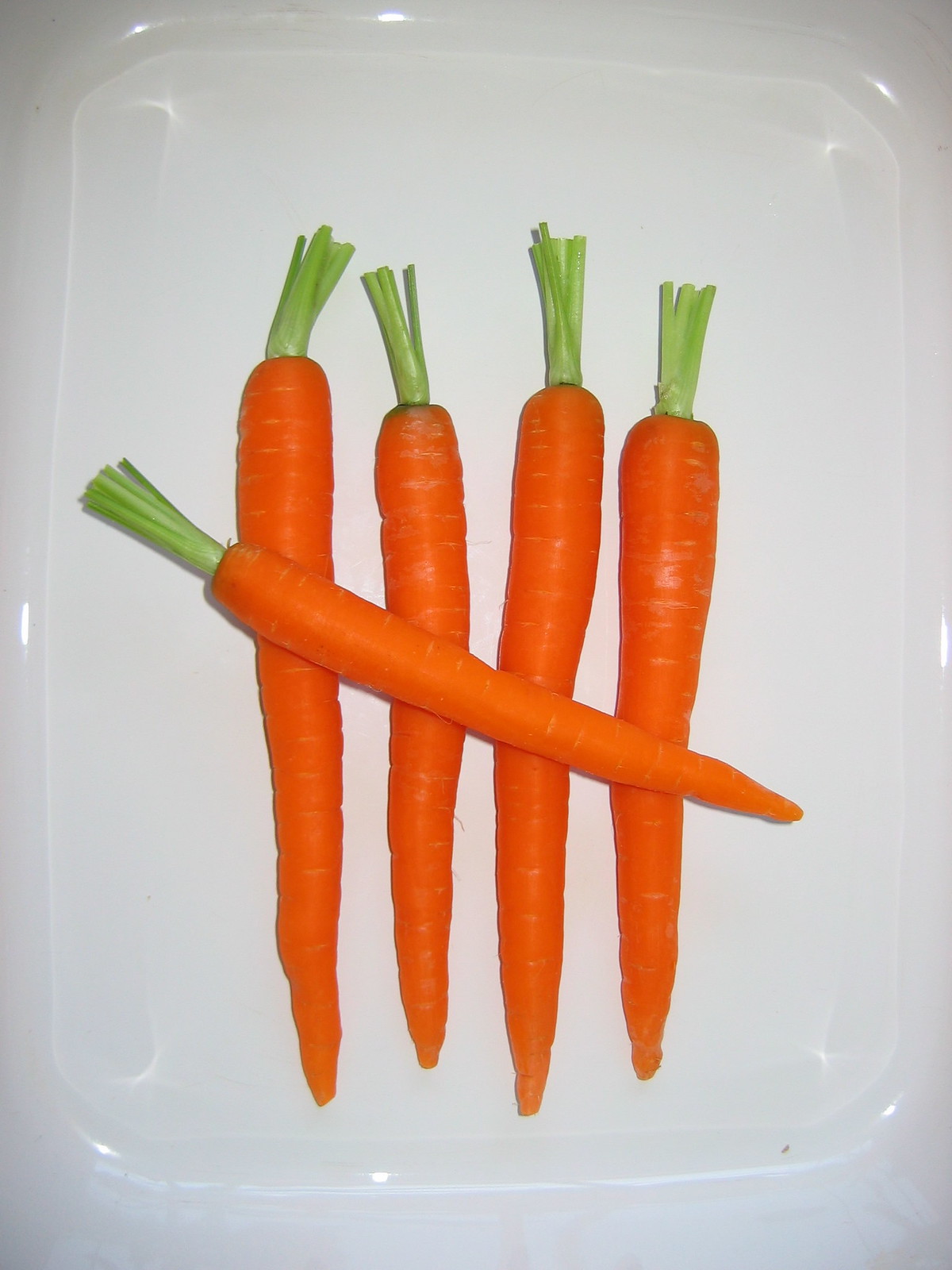The image is a detailed colour photograph, captured in portrait orientation, focusing on five bright orange carrots arranged on a white ceramic surface, likely a rectangular plate with rounded corners. Although the plate itself is not fully visible due to the tight crop, it reflects a bright light source, adding a subtle shine to its glossy surface. The arrangement of the carrots mimics the hash marks used in tallying numbers, with the points of four carrots arranged evenly, pointing downwards at a six o'clock position and their light green stems trimmed to about two inches, pointing upwards. The fifth carrot is placed diagonally across these four, with its green stem tilted slightly up to the left at a ten o'clock position, and its tip extending off the rightmost carrot at a four o'clock position. All carrots appear very uniform in size and color, displaying a smooth texture with some fine horizontal markings, and retain a moist, fresh appearance. The overall simplicity of the image, with its clean white background and bright hues, emphasizes the natural beauty and symmetry of the carrots.